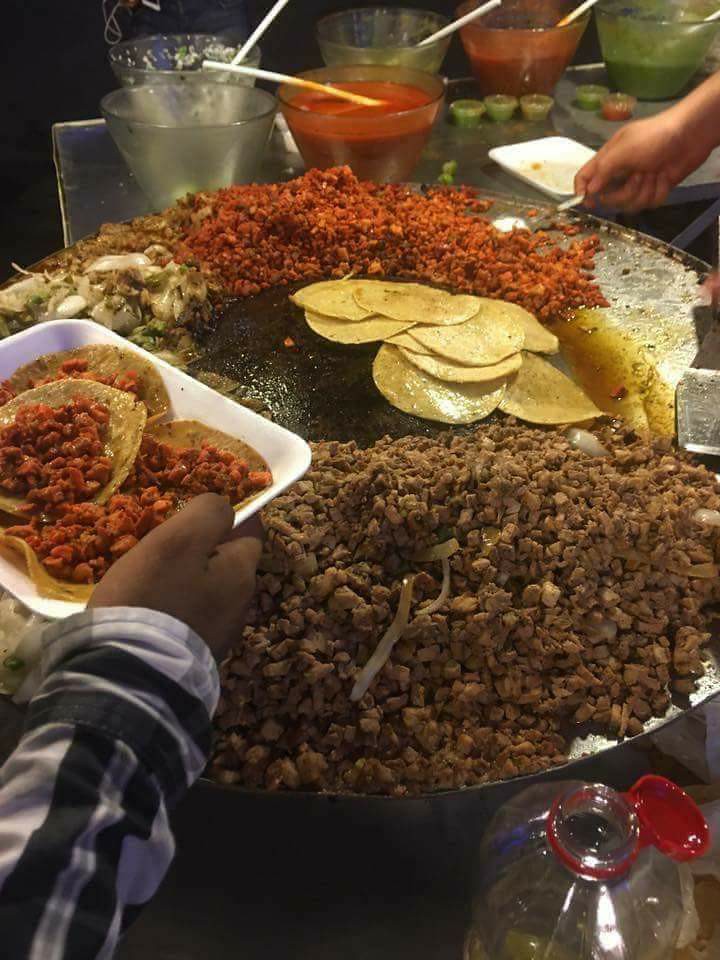The image depicts a bustling buffet scene centered around a gargantuan, circular silver serving platter loaded with an eclectic array of food. The platter dominates a gleaming stainless steel countertop, its slightly curved rim expertly containing the assortment of culinary offerings and their accompanying grease pools. 

A significant portion of the platter is crowded with chunks of ground-up chicken, visibly cooked to succulent juiciness, interspersed with a medley of both regular and green onions. Adjacent to this is a section of vibrant red, spice-coated chicken pieces, providing a stark contrast in color and hinting at robust, spicy flavors. Nestled within the center of this culinary display are numerous corn tortillas, several of which have absorbed so much grease that they appear almost soggy to the touch.

To the left side of the scene, a person’s right arm, clad in a white jacket with distinctive black stripes running along the middle and cuffs, is captured mid-action. This individual is holding a plastic tray with rounded edges, laden with three tortillas drenched in sauce until they turn brown. The tray also contains a modest assembly of beans and assorted vegetables like carrots.

In the background, one can distinguish a rectangular silver tray hosting various bowls filled with condiments, including salsa, mayonnaise, avocados, and a prominently placed jug of water, enhancing the dish’s versatility for different palates. Additionally, a hand extends into the frame, actively involved in scooping some unidentified morsels from the serving platter. This bustling and richly detailed scene conveys a sense of abundance and communal dining, possibly at a festive gathering or special event.